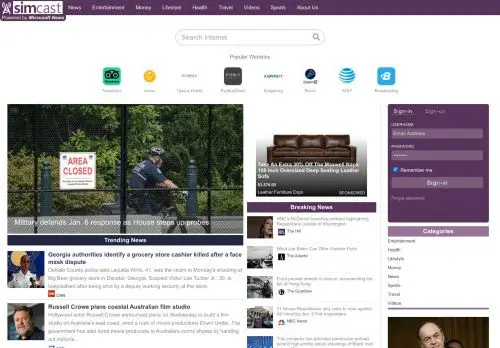Here is a detailed and cleaned-up descriptive caption for the image:

The image is a screenshot of a website that resembles a magazine layout, focusing on articles and news. This is the homepage of the site.

* **Banner and Navigation**: At the top, there is a dark purple bar spanning the width of the page. The website's logo, located at the top-left corner, appears to say "Simcast," accompanied by an icon resembling a radio tower emitting signals. To the right of the logo is the navigation menu, containing approximately eight items, though the text is too small to discern from this image.

* **Search and Popular Websites**: Directly below the navigation bar, in the top center, is a search field labeled "Search Internet." This search bar is white with rounded ends and includes a magnifying glass icon on the right. Below the search bar is a section labeled "Popular Websites," featuring eight icons in a horizontal row. Starting from left to right, the first icon is recognizable as TripAdvisor. The second icon is gold-colored and might represent Volkswagen, although the color does not match Volkswagen's typical branding. The third icon is mostly unreadable, presenting black text on a white background. The fourth is a black square with small white text. The following four icons include AT&T as the second to last recognizable one, and the last icon appears to be a blue square with a white "b."

* **Main Content Area**: The main content is divided into three columns on a white background.
  
  * **First Column**:
    * The largest column featuring a prominent image of a person dressed in black and wearing a helmet, standing behind a black chain-link fence with a sign that reads "Area Closed" in red letters. There is also some overlay text on the image that is mostly unreadable but seems to reference a "January 8th response."
    * Below the image is a blue bar labeled "Trending News," presenting two articles with thumbnail images and excerpts. One article includes a close-up portrait of a man with the headline seemingly mentioning Russell Crowe and an issue related to film audio.
  
  * **Second Column**:
    * The top image depicts a brown leather sofa in a white room. It has some overlaid text that is unreadable. Below this image is a purple bar labeled "Breaking News." This column lists five articles, each with a thumbnail image, a headline, and an excerpt.
  
  * **Third Column**:
    * This column, slightly smaller than the second, features a purple box at the top with options to "Sign In" and "Sign Up," followed by corresponding input fields. Below this is another purple bar with unreadable text, followed by a column of text cut off due to the image's end.

Overall, the website layout is informative, visually structured, and focuses on categorizing various articles and search functionalities for visitors.